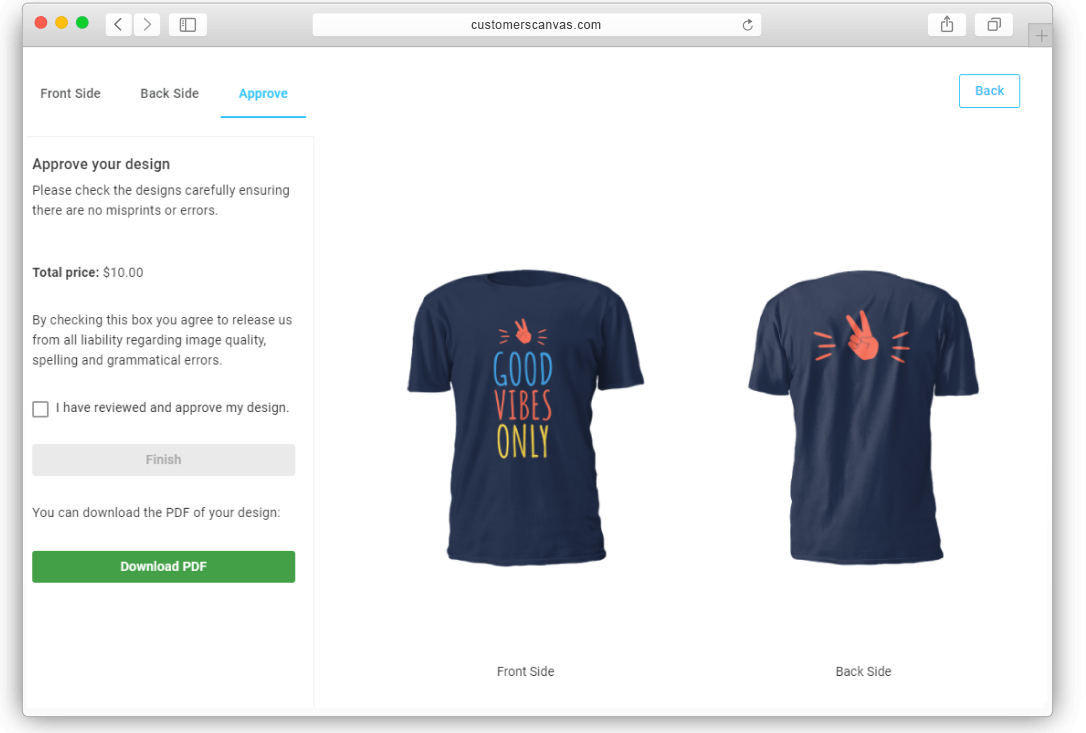**Detailed Caption:**

The mock-up showcases a website being viewed in an Apple browser, characterized by the distinctive red, yellow, and green buttons at the top left for closing, resizing, and maneuvering the window. The browser's address field displays "Customers, Canvas.com" alongside the forward and backward navigation options. 

Below this, the main website interface features a series of options including "Front," "Side," "Back Side," and "Approve," with the "Approve" option underlined in blue. To the right, a prominent "Back" button is visible. 

A section titled "Approve Your Design" prompts users to carefully inspect the designs for any misprints or errors. Below this message, the total price is stated as $10. An informational disclaimer requires users to agree to release the service from all liability concerning image quality, spelling, and grammatical errors, and includes an unchecked checkbox labeled "I reviewed and approved my design."

The interface also features a light gray button labeled "Finish," which users can press to complete their actions. Additionally, there is an option to download a PDF of the design via a green button labeled "Download PDF."

To the right, the mock-up presents two images of a slate blue t-shirt, displaying both the front and back sides. The t-shirt's front features a peace sign with three dynamic marks emanating from it, accompanied by the text "Good Vibes Only." The words "Good" and "Only" are in a hand-drawn, all-caps, simple font, with "Good" in blue, "Vibes" in orange matching the peace sign, and "Only" in yellow. The back side of the t-shirt showcases the same peace sign logo without any accompanying text.